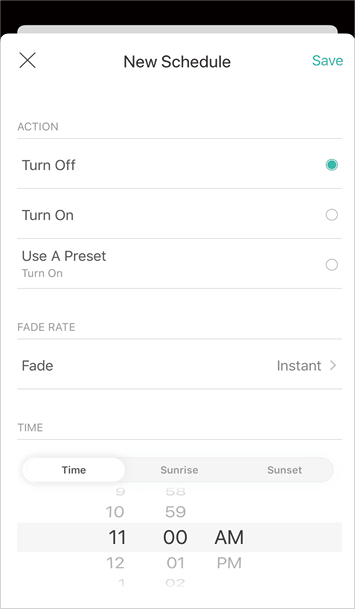The image displays a digital interface for setting a new schedule, prominently featuring the heading "New Schedule" at the top. The word "Save" is highlighted in light green, indicating an option to confirm the settings. Below the heading, there is an action button accompanied by a light line, labeled "Turn Off," represented by a solid turquoise circle. Additionally, there is an option for "Turn On," shown as a clear circle, and "Use a Preset," also depicted with a clear circle. 

Each option is followed by a light gray line to separate them visually. The interface further includes settings for "Use a Preset," with another light gray line, and "Fade Rate," also highlighted by a light gray line leading to a subsection where "Fade" and "Instant" options are illustrated with a right-pointing arrow. This section ends with a gray line.

Beneath this, the interface allows scheduling by time, marked by another gray line. Users can select specific times, sun events like "Sunrise" or "Sunset," and choose between a.m. and p.m. options through a scrolling menu. This entire configuration area is encased within a white box, bordered by a gray line, and the interface is framed with a black border at the top. An 'X' icon indicates an option to close or exit the scheduling interface.